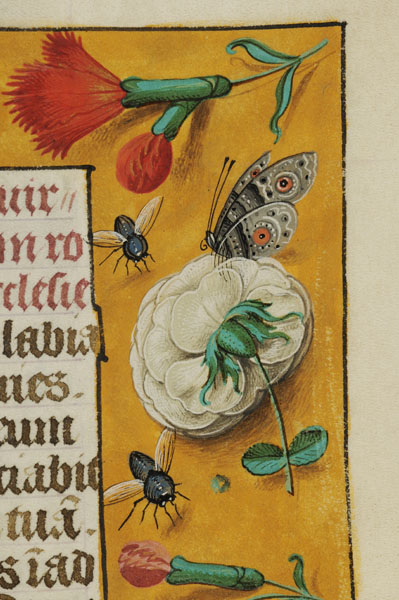The image presents a detailed segment of artwork, possibly from an illustrated medieval manuscript or ancient book, covering approximately 25% of a larger piece. A grayish cream border frames the artwork from the top left to the bottom right, tapering off towards the other edges. The inner background features a goldish-yellow hue with a slender black line outlining it. There is also a rectangular section containing text in a non-English language, possibly Latin, bordered in black. The text, written in red and black ink with little grey lines, is only partially visible and appears to be cropped.

Within this ornate setting, various flora and fauna are illustrated. A prominent white flower with a green stem and a red flower with green leaves stand out. Among the fauna, several insects are depicted, including black flies with clear wings, bees, and a gray butterfly adorned with orange eye-like spots on its wings. Additionally, an orange leaf and flower extend from a green stem near the top, and a yellow-white flower is also present. The entirety of this piece is rendered with meticulous detail, evoking the intricate style of medieval monks.